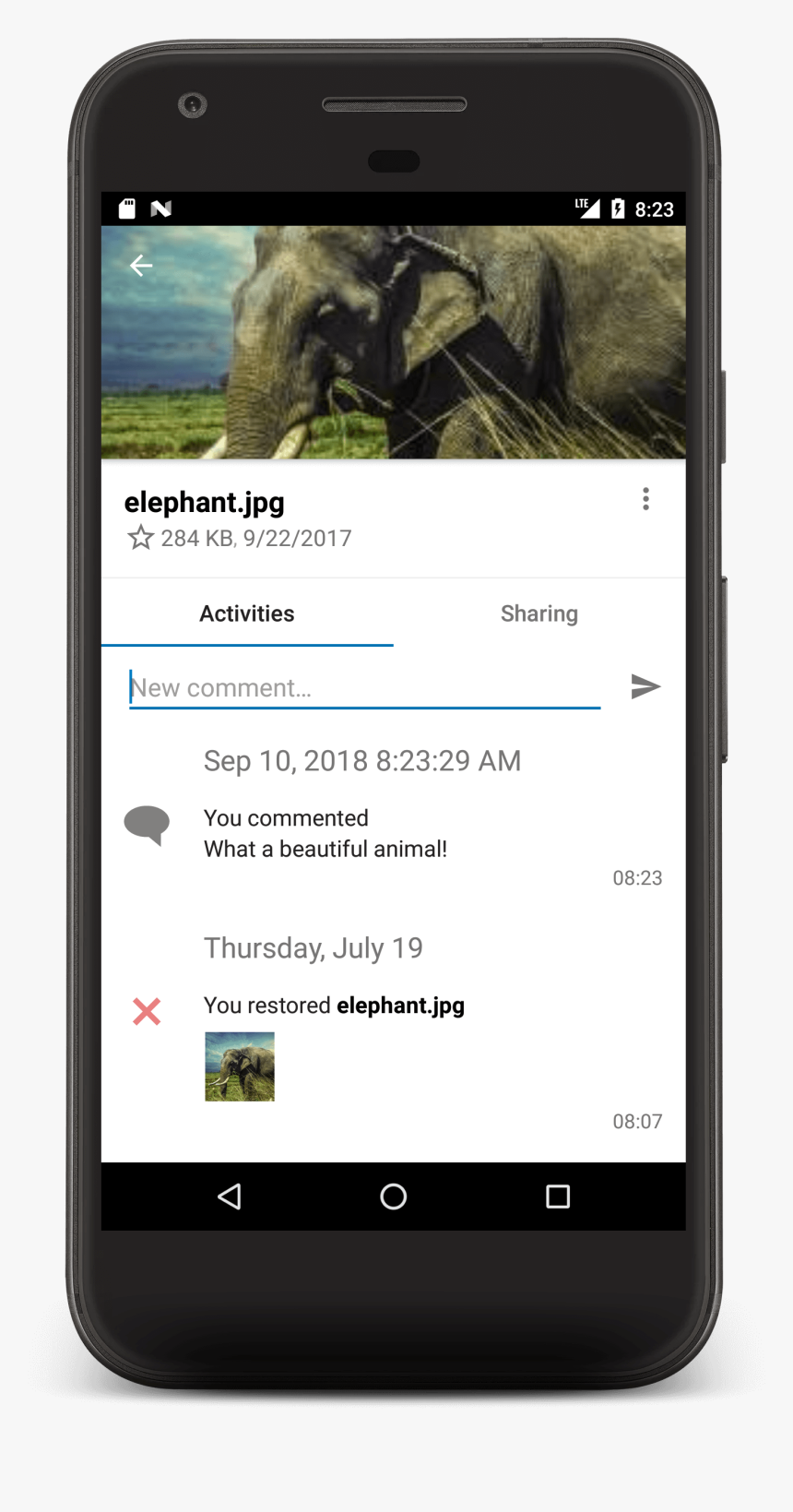A black mobile device is depicted in the image, showcasing its various design elements and functionalities. The camera is positioned in the upper left corner of the device, while a speaker grill is centrally located at the top, with a sensor positioned just beneath it. The power button is situated on the top right side of the phone, and the volume up and down buttons are located in the right center section.

On the phone's screen, a thin black bar at the top serves as the notification area, indicating that the SD card has been removed, the battery is currently charging, and the time is 8:23. The main screen displays a picture of an elephant in a field, titled "elephant.jpg." Details about this image include its size (284 kilobytes) and its date (September 22, 2017). A back arrow is present at the top section of the image.

Below the picture, there are tabs for "Activities" and "Sharing," followed by a section for new comments and a button to send comments. Existing comments are displayed underneath, where one reads, "You commented: What a beautiful animal." Another entry shows that on Thursday, July 19th, the user restored the file named "elephant.jpg."